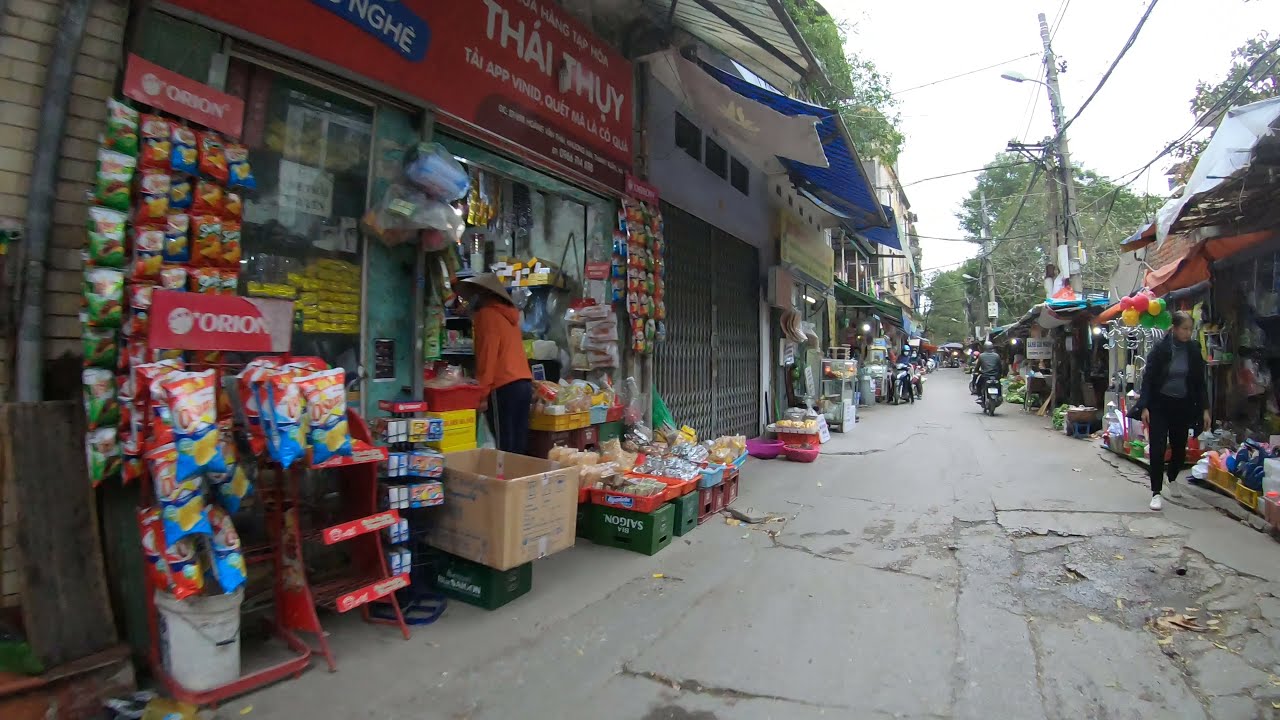In this horizontally aligned rectangular image, we see a bustling street scene in what appears to be Thailand, evidenced by the storefront sign "Thai Thui." The street is narrow and lined with small shops and market stalls, each displaying a variety of goods such as bags of chips, hanging on hooks, and stacked on shelves. The road itself is in poor condition, with numerous cracks, holes, and uneven patches most visible in the lower right corner. In the lower left corner, a slightly blurry stall outside a store bears the sign "Orion," showcasing numerous snack bags. 

A person in an orange hoodie, black pants, and a sombrero-like hat stands near this stall, peering into the store window. Across the street, there's an array of quaint, shack-like shops, also filled with products outside their doors. In the distance, several motorcycles can be seen, including one with a rider moving away. The scene also includes a lady dressed in dark clothing walking towards the camera on the right side, seemingly engrossed in the street vendors' offerings. Above the shops and street, a tangle of power lines stretches across the scene, with glimpses of bright white sky peeking through on the upper right side, accentuating the lively but aged character of this street.